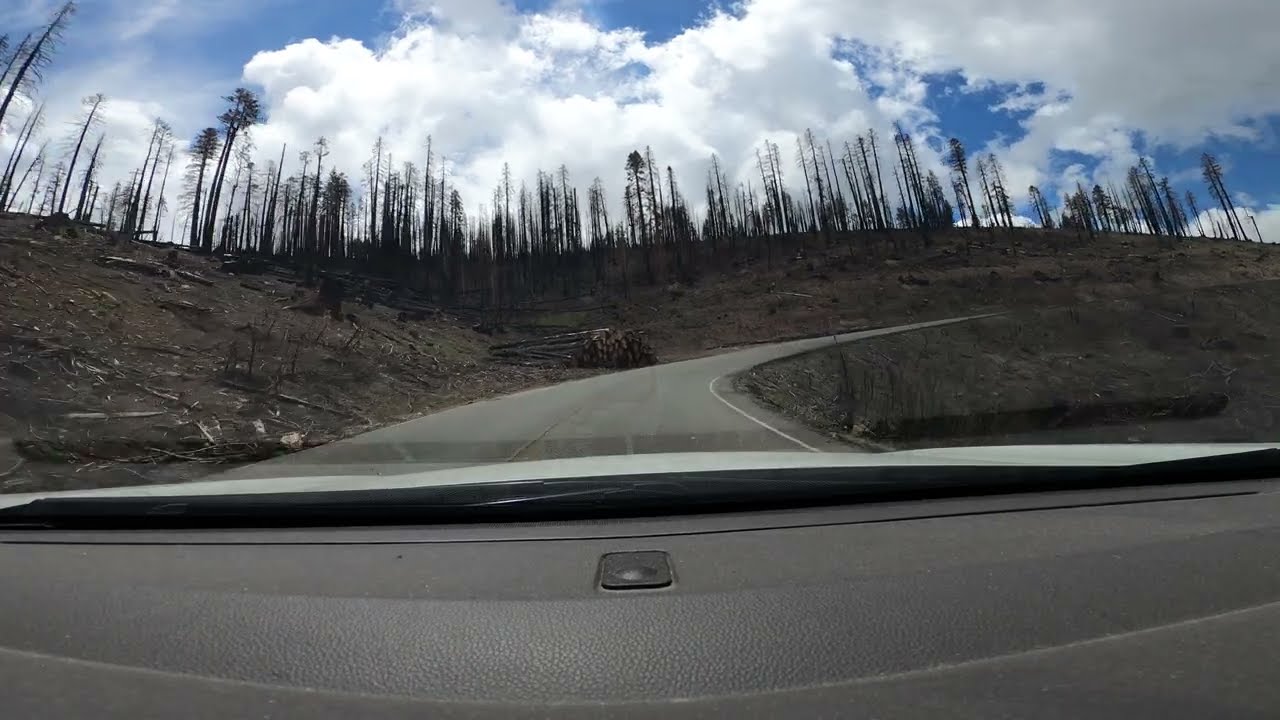This image captures a panoramic view from the inside of a car, looking out through the front windshield. Dominating the bottom of the frame is the dark gray dashboard of the vehicle, partially obstructing the view of the white hood and a visible windshield wiper. Ahead, the road curves gently to the right, framed by a hill on the left side that follows the same trajectory.

The landscape along the sides of the road is sparse and rough, characterized by tall, slender, and scruffy-looking trees, many of which have been cut down or appear to have been burned, with some still standing but looking largely unhealthy and bare. Piled near the road is a stack of logs, neatly arranged, evidence of recent logging. The roadside to the right shows signs of brush and other undergrowth.

The overall scene is under a sky dotted with large, puffy white clouds, which are interspersed with patches of bright blue. The clouds stretch across the entire horizon, creating a striking contrast against the otherwise brownish and sparse landscape. The forested hill and broken, irregular patches of tree cover add to the rugged and desolate feel of the environment.